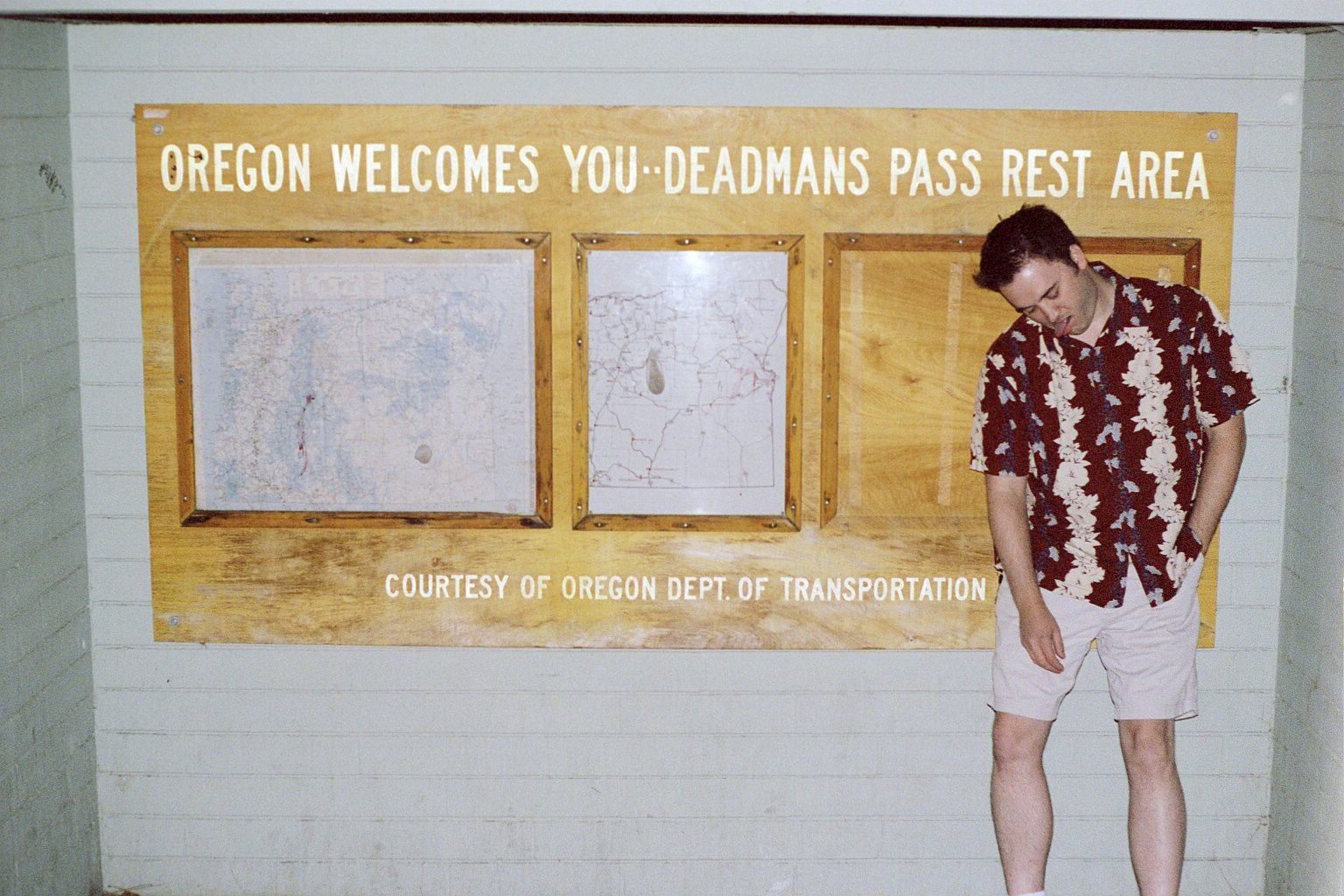In this image, a man in his 20s or 30s with black hair is posing playfully with his tongue out in front of a sign at a rest stop. He is wearing a vibrant red and yellow Hawaiian-style shirt and khaki shorts. The sign, which is mounted on a white brick wall, reads "Oregon welcomes you, Dead Man's Pass Rest Area, Courtesy of Oregon Department of Transportation." The sign consists of three framed sections; two of them contain maps, presumably of Oregon, while the third frame is wooden and contains the text. The rest stop’s wall has a wooden panel motif with illustrations that resemble windows, adding to the aesthetic of the display. The man seems amused by the "Dead Man's Pass" designation and is making a face as if he were playing dead, capturing a lighthearted, touristy moment.